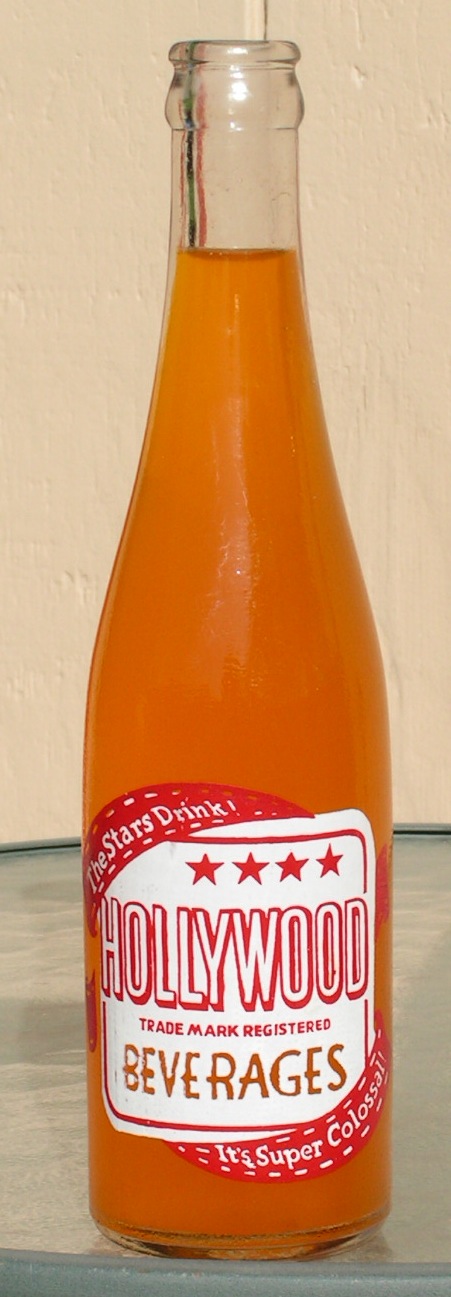The photograph depicts a tall, slender bottle of an opaque, medium-light orange beverage, prominently positioned against a pale pink masonry wall. The bottle rests on a light gray counter, indicating it has been opened as it lacks a lid. The beverage within the clear bottle appears somewhat thick in consistency, making it non-transparent. The bottle features a distinctive white, square label with reddish-pink lettering and a golden embellishment. The label reads "The Stars Drink" at the top, followed by four stars. Below this, "Hollywood" is inscribed in block letters, and beneath that, the text "Trademark Registered Beverages" is displayed. At the bottom of the label, the phrase "Super Colossal" is prominently written, highlighting the beverage's substantial and impressive nature.